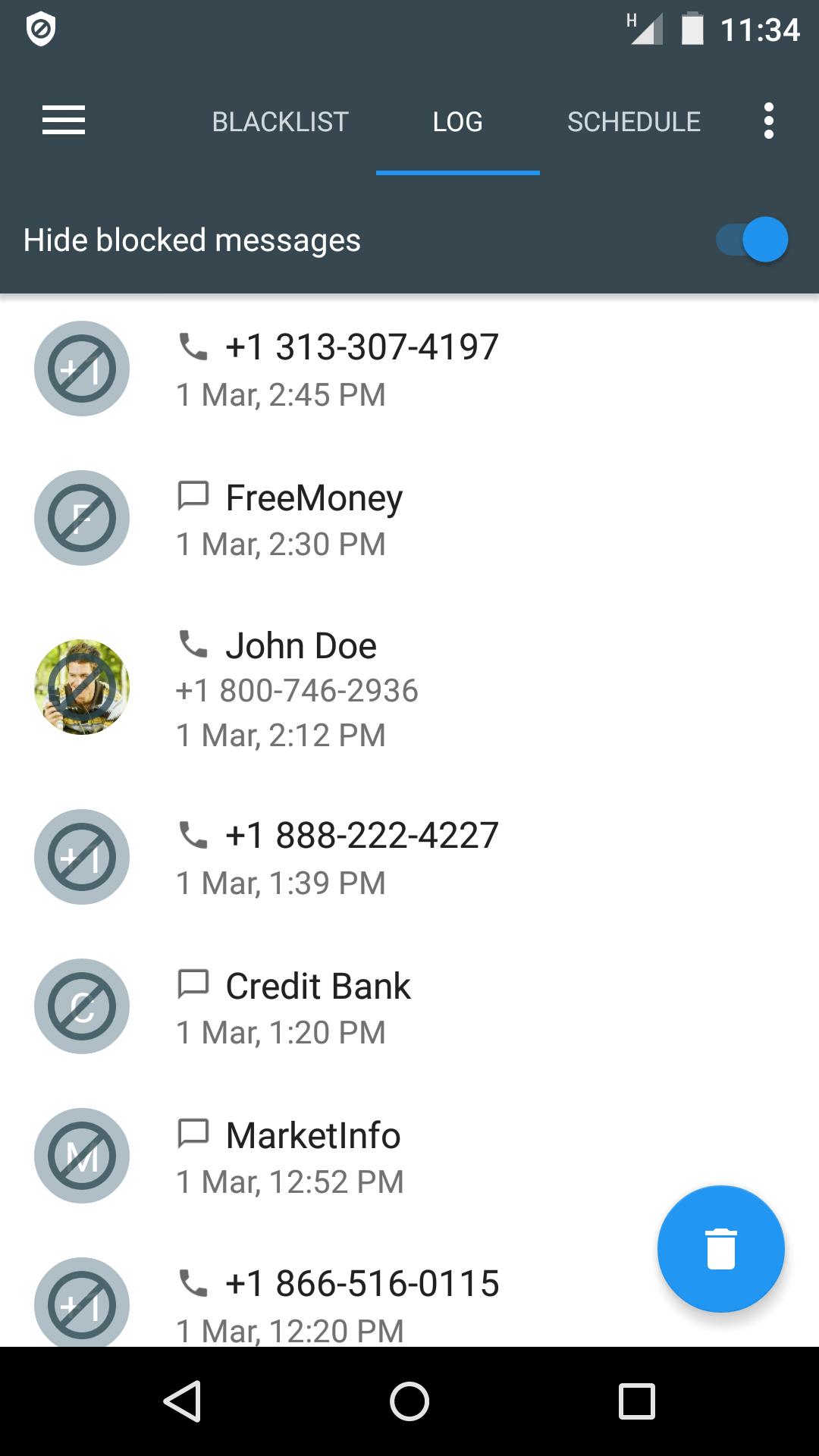**Detailed Caption:**

This image features a screenshot of a mobile device displaying a call log interface with a predominantly white background. The upper portion of the screen has a black rectangular background housing a menu bar. At the top left, there is an antivirus icon, followed by indicators that show a moderate network signal and a fully charged battery. The time displayed is 11:34. 

On the same menu bar, from left to right, there are icons including a hamburger menu, "Blacklist," "Log," "Schedule," and another hamburger menu. The "Log" tab is highlighted with a blue underline. Below this row, there is an option labeled "Hide Blacklisted Messages," accompanied by toggle switches to turn the feature on or off.

The main section of the screen presents a call log styled interface with seven entries, each featuring contact information and corresponding icons. Most icons are placeholders with symbols that include a null signal (a circle with a slash). The third entry, however, features a stock photo of a man.

The call log details are as follows:
1. A call from a 313 area code number on March 1st at 2:45 PM.
2. A text message from "Free Money" on March 1st at 2:30 PM.
3. An 800 number labeled "John Doe," likely a scam, on March 1st at 2:12 PM.
4. A call from an 888 number on March 1st at 1:39 PM.
5. A text from "Credit Bank" on March 1st at 1:20 PM.
6. A text from "Market Info" on March 1st at 12:52 PM.
7. A call from an 866 number on March 1st at 12:20 PM.

At the bottom of the black rectangular section is a call button and a go-back button.